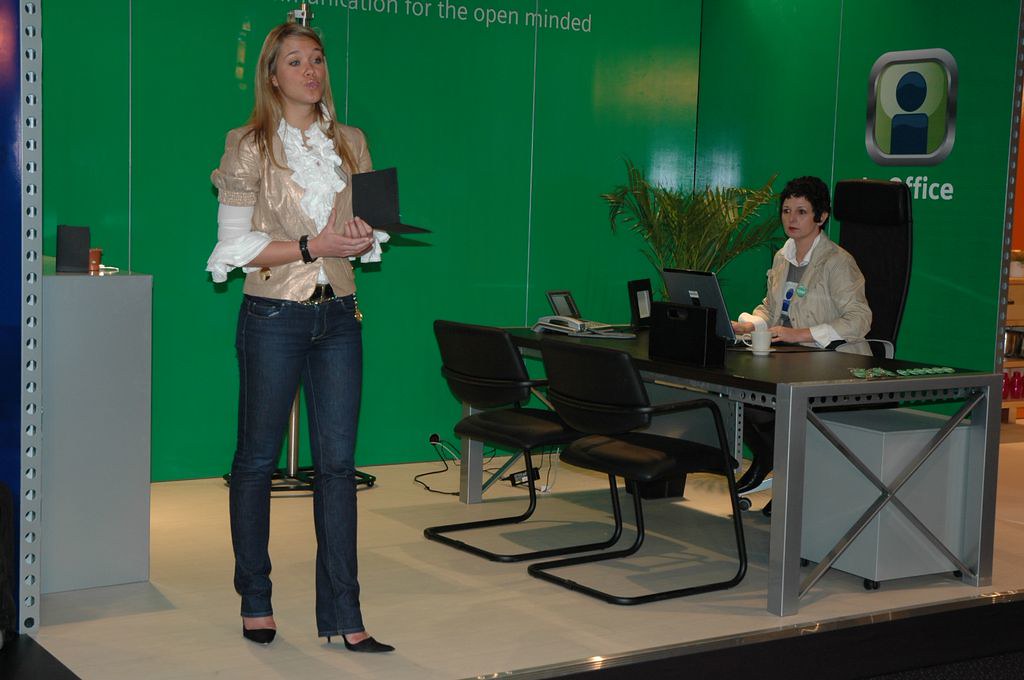In this photograph of an office space, two women are featured prominently. The standing woman, who has blonde hair and light skin, is wearing a stylish outfit consisting of a white frilly designer shirt beneath a shiny gold lamé vest, blue jeans, and black high heels. She also has on a black watch and is holding a black book while looking straight ahead. The woman standing near her sitting colleague, whose light skin and dark curly hair contrast with her tan jacket and white collared shirt. This seated woman is positioned at an industrial-style desk made of gray and black metal with a laminate finish. In front of her, the desk features a laptop, a cup of coffee, a black landline telephone, and various other items. Two black steel chairs with black cushions are positioned in front of the desk, while a large green palm plant adds a touch of nature in the background. The walls of the office are a dark, shiny green with a logo that emphasizes open-mindedness. The floor is tan-colored, and a gray cabinet with a black rectangle and a red rectangle on it is placed across from the standing woman.